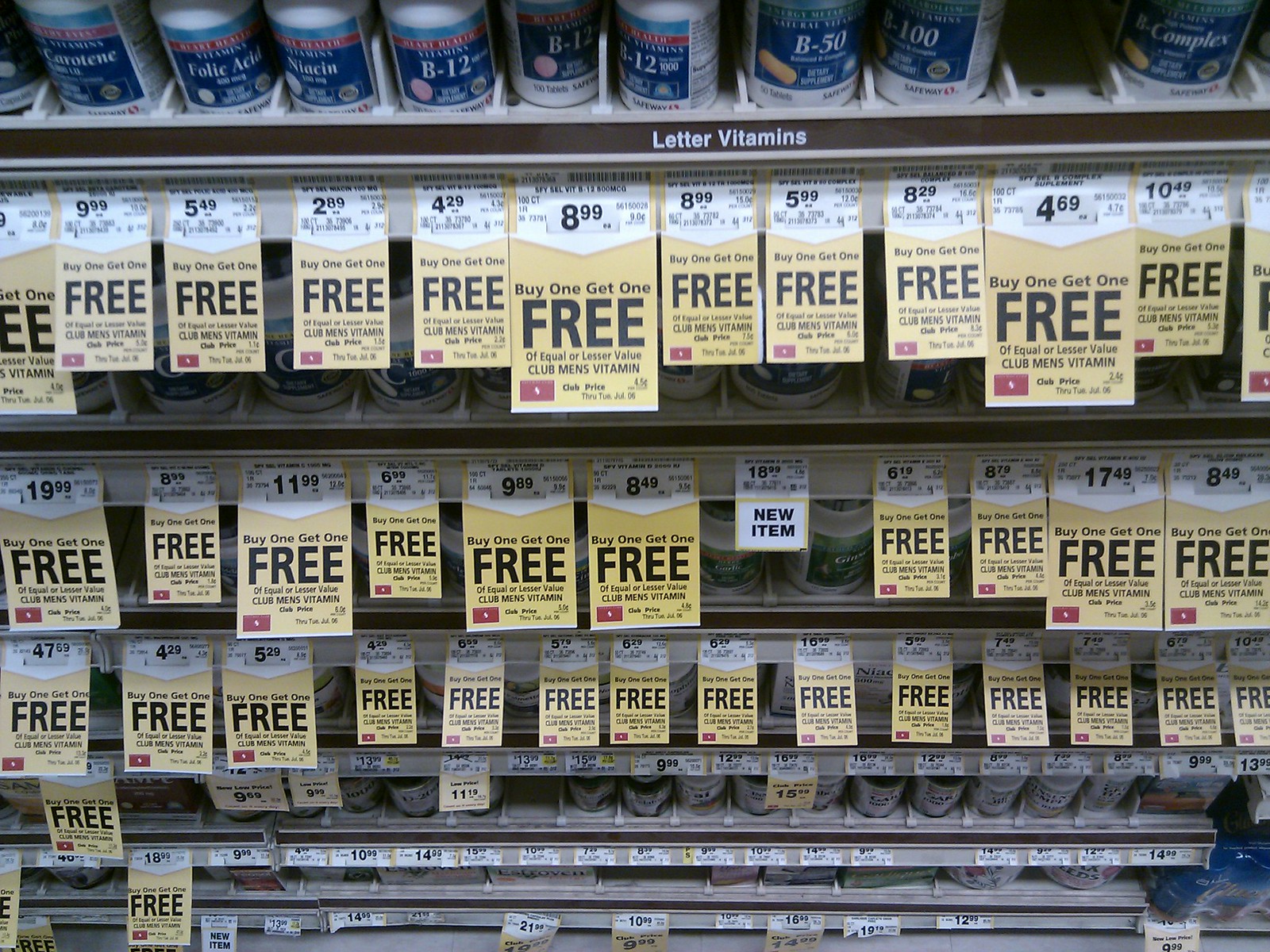The indoor color photograph captures a close-up view of a vitamin display in a drugstore. The display consists of multiple vertical shelves, approximately seven or eight in number, each densely packed with various vitamin bottles. Prominently visible are vitamins such as B50, B12, folic acid, niacin, B100, and B-complex. Each shelf is lined with numerous rectangular price tags, around 20 to 30 in total, which prominently feature a "Buy One Get One Free" promotion. The price tags are white with the promotional message in a contrasting yellow field, stating "of equal or lesser value" below the offer. The tags are so large that they partially obscure the bottles behind them, emphasizing the store's significant sale event. This detailed arrangement highlights the vibrant and busy aesthetic of the retail display.